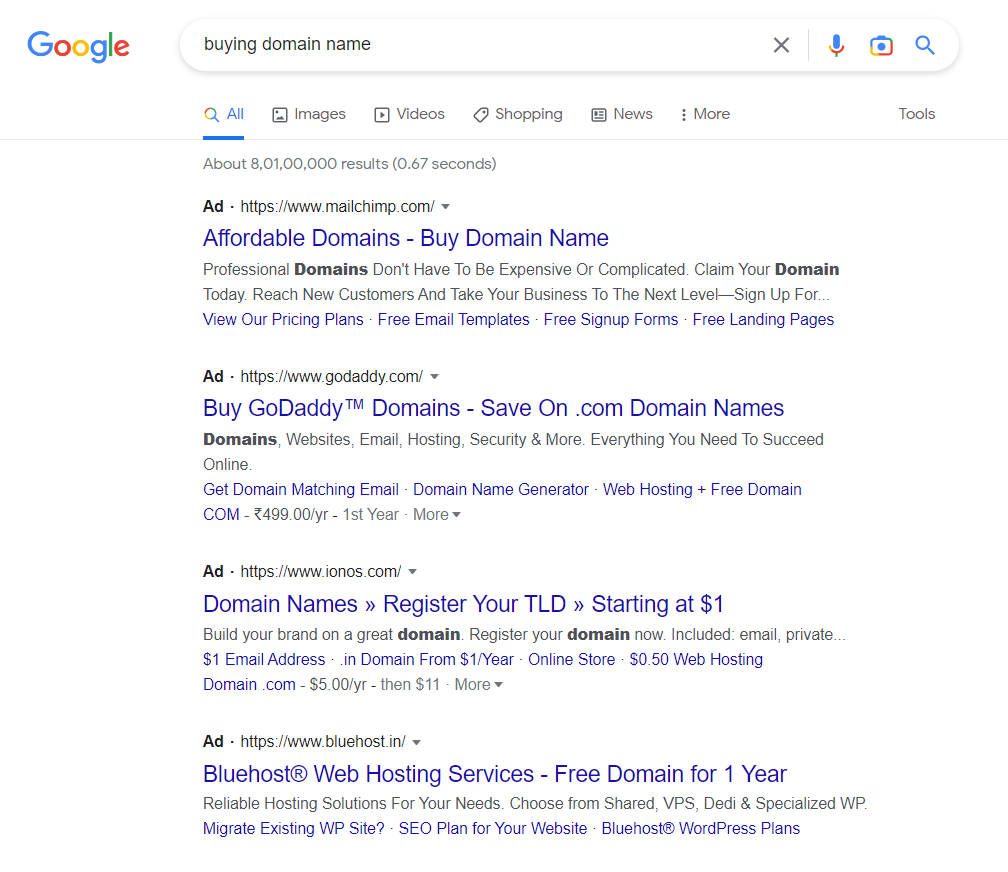The image shows a Google search results page with a white background. In the top-left corner, the colorful "Google" logo is prominently displayed. Adjacent to the logo is an oval search bar containing the query "buying domain name." To the right of the search bar are four icons: an 'X' for clearing the query, a colorful microphone for voice search, a colorful camera for image search, and a blue magnifying glass for initiating the search.

Below the search bar is a horizontal menu with various tabs, including "All," "Images," "Videos," "Shopping," "News," and "More." To the far right of this menu, there's a "Tools" option. 

Below this menu, the search results are summarized with an indication of about "8,01,00,000" results, which appears to be a typo for 8,000,000 results. Under this summary, there is a selection of clickable links, all marked as ads. The ads are related to domain name purchases and web hosting services, featuring companies such as GoDaddy and Bluehost, along with descriptions like "affordable domains" and "buy domain name."

Each ad provides a brief overview before clicking through for more details.